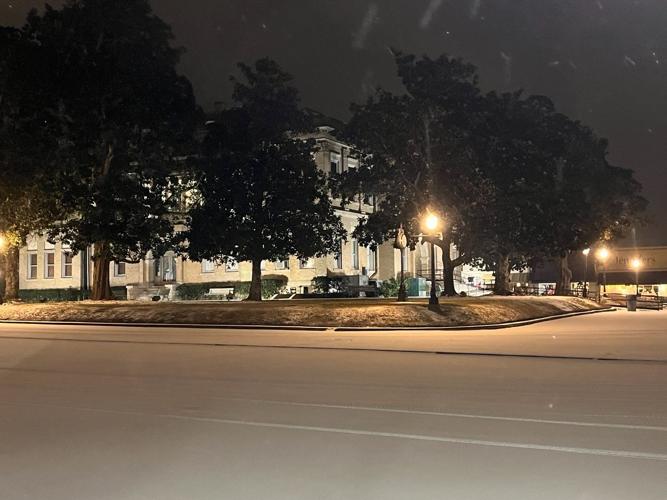A blurry nighttime scene captures a large, illuminated office building partially shrouded by tall, dark trees, including deciduous varieties and a pine tree. The two-story structure, with white to yellow walls, stands on a corner, and features multiple windows and two entranceways. The building's silhouette is highlighted by streetlamps lining the roadway in front, which is devoid of cars and people, suggesting it was taken in the very late or early hours. The road has clearly visible white lane markings and a guardrail or fence along its edge. Faint text, possibly indicating "Jennifer's," is visible on a sign to the right of the image. Bushes around the building are neatly trimmed, and two benches can be seen among the vegetation. Behind the main building, another structure, possibly a parking facility, is discernible. The overall scene is dominated by dark tones, with the gray of the building, the night sky, and the subtle illumination lending an ambient glow to the setting.